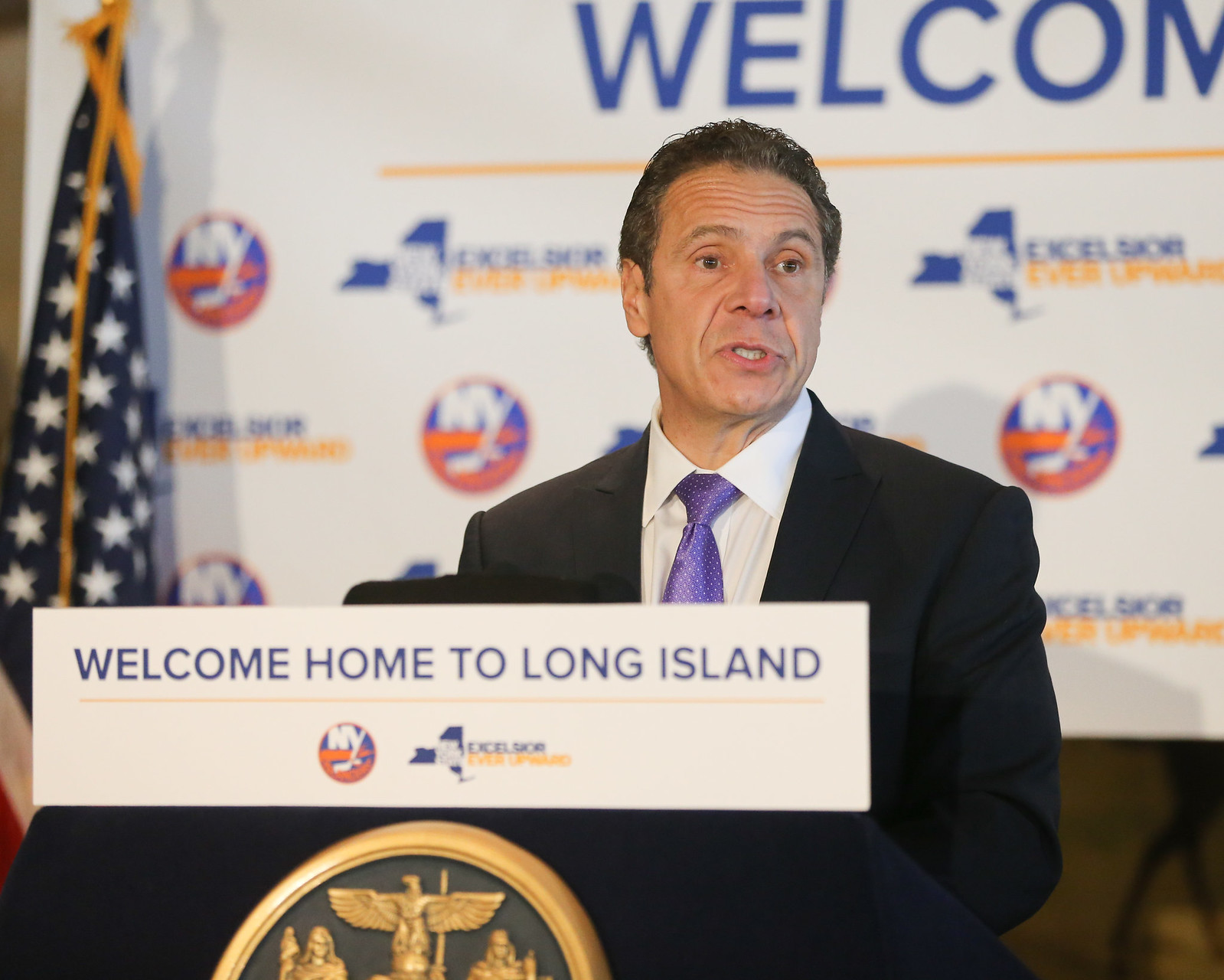In this detailed photograph of a press conference featuring Governor Cuomo of New York, he is positioned centrally, standing at a podium adorned with a gold-emblemmed seal and a sign that reads, "Welcome to Long Island." The podium also features the New York Islanders logo and the word "Excelsior" beneath it. Governor Cuomo is attired in a dark suit, a white button-down shirt, and a purple tie with white dots. Behind him hangs a large banner emblazoned with the word "Welcome," accompanied by various icons including the New York Islanders logo and a depiction of the state of New York. To the left of the image, an American flag with gold fringe and tassels is prominently displayed. The indoor setting, likely a convention hall, adds to the formal atmosphere of the event.